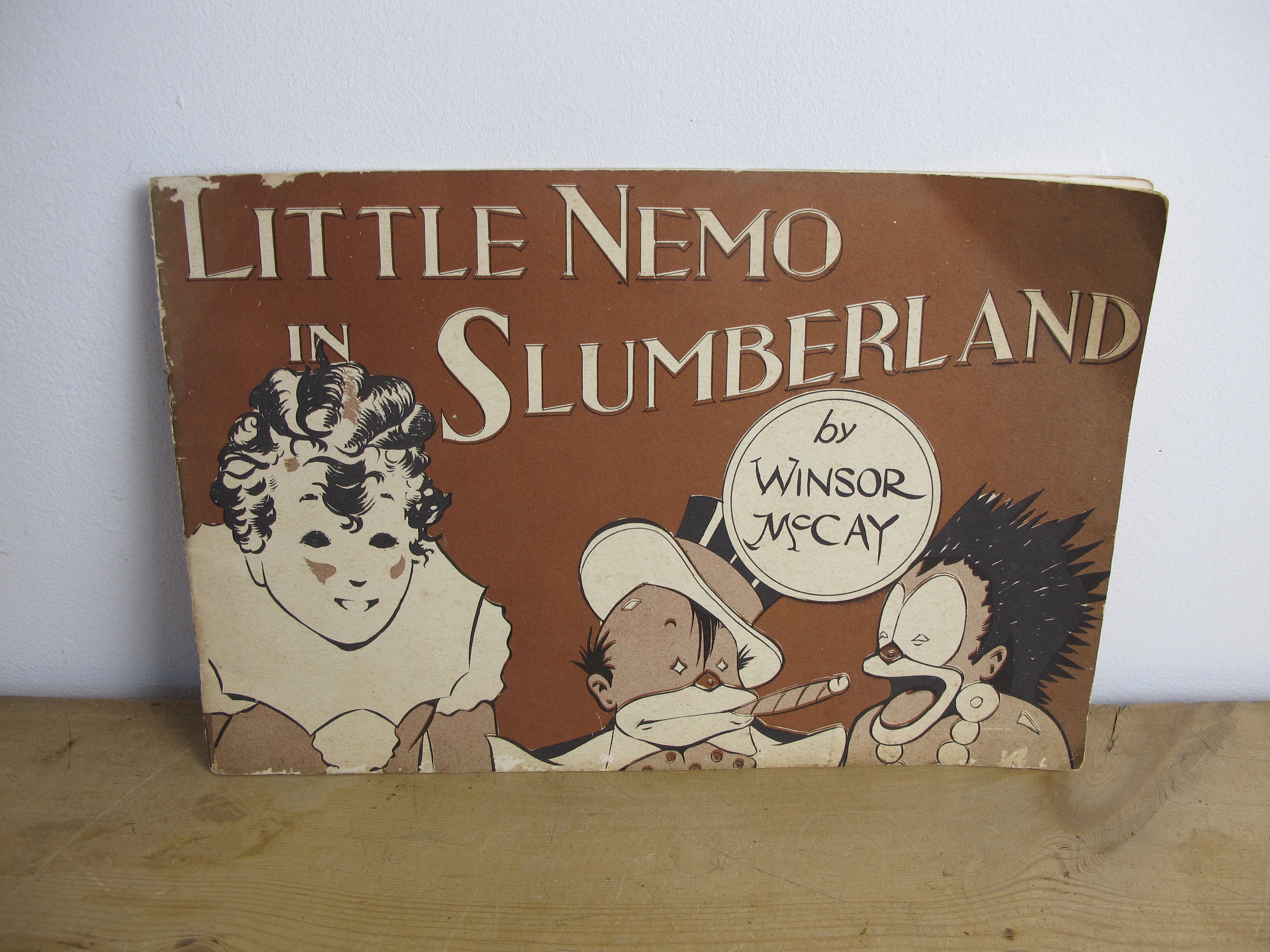The image shows an old children's book titled "Little Nemo in Slumberland" by Winsor McCay, likely dating back to the 1920s or 1930s. The book features a distinctively horizontal, softback cover, primarily colored in browns, blacks, and whites. It is placed on a wooden surface, leaning against a whitewashed wall, and bathed in natural sunlight.

The cover art is quite detailed and whimsical, with a central theme of caricatures. At the top, the large white text spells out the title against a brown backdrop. Below this, three prominently exaggerated characters are displayed. On the left side, there is a figure resembling a girl with Shirley Temple-like curly short hair, dressed in what appears to be a clown costume. The middle character is a man wearing a top hat and smoking a cigar, signifying wealth; he has exaggeratedly large lips and a red nose. On the right, another figure with similarly exaggerated lips and a red nose appears shocked; his bright, spiky hair sticks straight out as if electrocuted, and his mouth is wide open. These elements give the book a captivating, fantastical appearance, reflecting its dreamlike content.